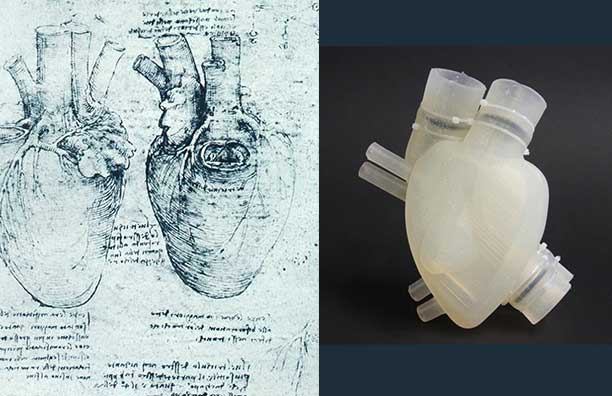The image is a detailed side-by-side comparison. On the left side, there is an ancient-looking, anatomical drawing of two views of a human heart from an old textbook. The paper appears aged, with unfaded pages containing written notes that are too small and indistinct to read. The heart drawing displays the main blood vessels emanating from it. On the right side, there's a photograph of a white, plastic prototype resembling an artificial heart. This modern-looking device has connections and openings, indicative of a scientific model possibly used for transplants. The plastic heart is set against a blue and black background, highlighting its clinical design in contrast to the historical depiction on the left.